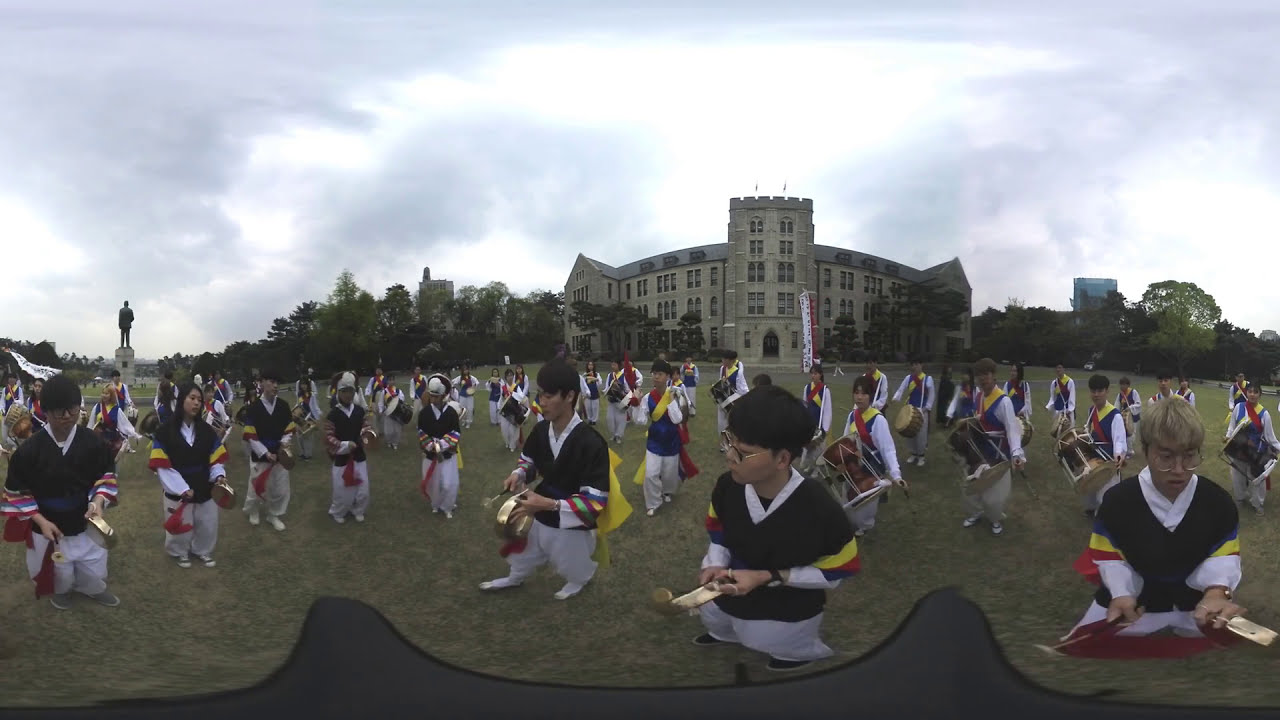The photograph captures a vibrant outdoor event taking place on a green field in front of a light brown university building that spans three to four floors. Under a blue sky with scattered clouds, numerous Asian students are participating in what appears to be a traditional cultural dance or musical ceremony. The students are dressed in black shirts with colorful patterns on the sleeves, white pants, and white shoes, and they are holding musical instruments that add to the festive atmosphere. The scene is meticulously organized, with the participants standing in a choreographed manner, possibly practicing or performing a routine. To the left side of the photo, there is a statue, adding a touch of monumentality to the scene. The image appears slightly curved, as if a fisheye filter or panoramic technique has been used to capture the wide expanse of the field and the detailed backdrop of the building and trees.